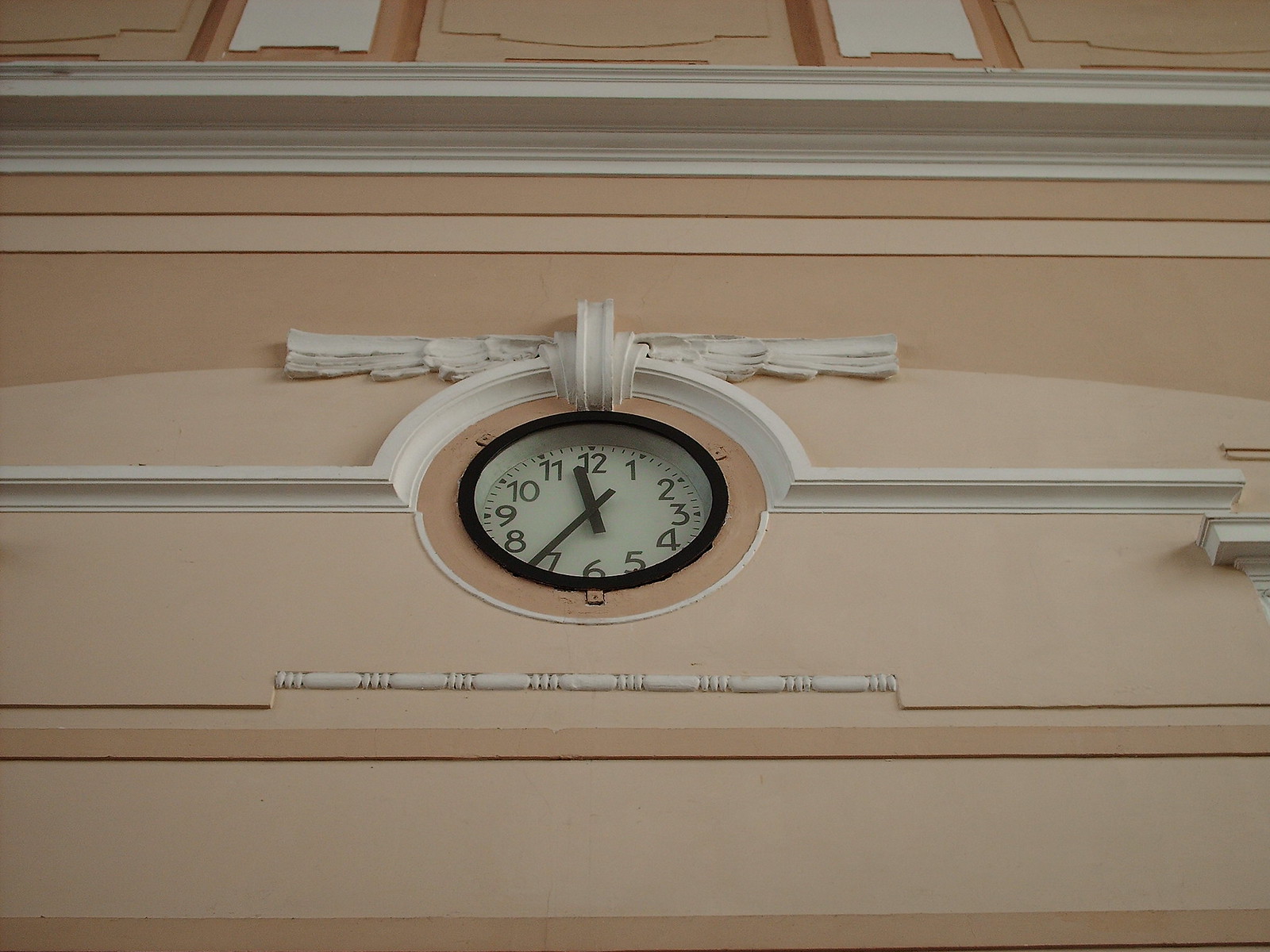The image captures an upward view of an intricately designed indoor wall that is a mix of beige, light brown, and peach, creating a light orange hue. The wall features horizontal white bars and faceted elements that add depth and texture. Centrally embedded into the wall is a round clock with a white face and black circular frame. The numbers and hands on the clock are thick and black, giving it a bold and basic appearance. The clock, displaying the time just after 11:35, sits high on the wall. Above it, a decorative white design resembling a bow adds a touch of elegance, while beneath it, an etched pattern provides additional detail. To the top of the image, two areas that look like windows with shutters or framed squares in white and peach can also be seen. On the right side of the wall, pillars add to the architectural interest of the scene.